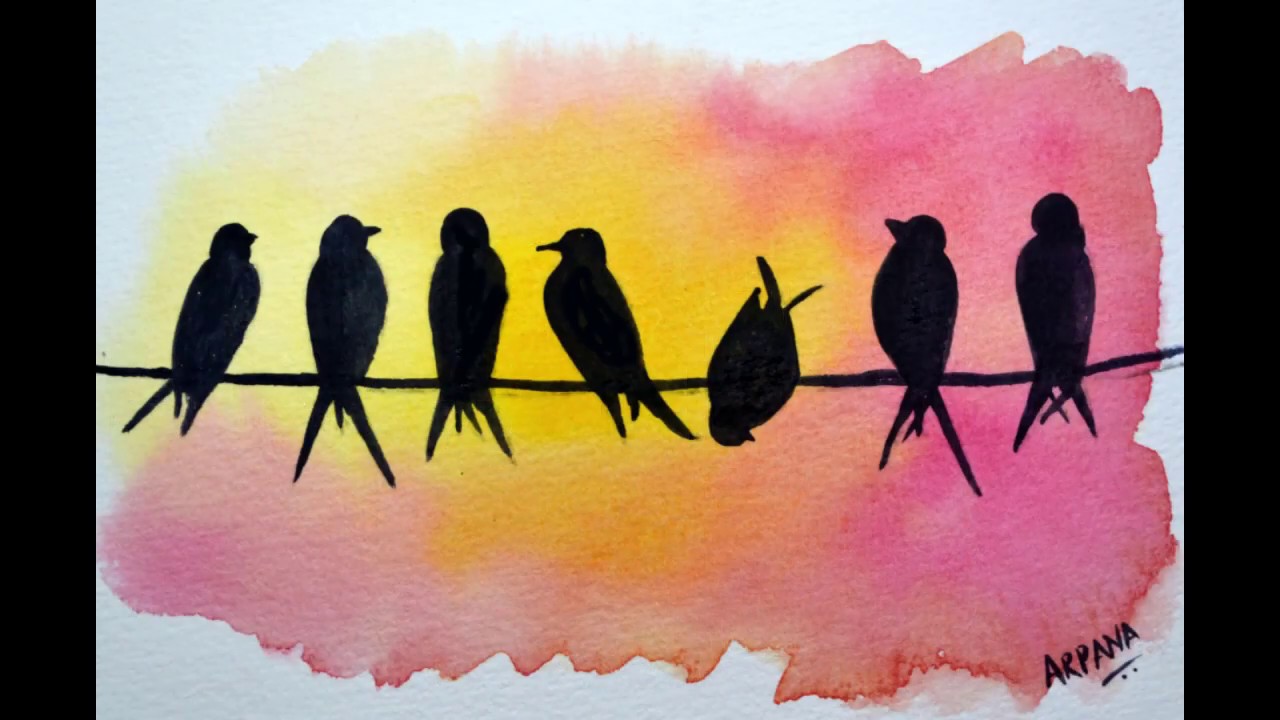The image is a watercolor painting of seven blackbirds perched on a telephone wire against a dreamlike sunset. The gradient sky transitions from yellow at the center to pink and orange, evoking an afternoon sun setting. Most of the birds are upright, facing various directions, while one bird, the third from the right, hangs upside down as if it just landed or is about to fall. The fourth bird from the left is in profile, facing the viewer's left. The artwork features the signature "ARPANA" in the bottom right corner, accompanied by a distinctive marking with a slash and two dots underneath. The painting appears slightly blotchy, indicating it may have been painted with wet watercolor techniques.